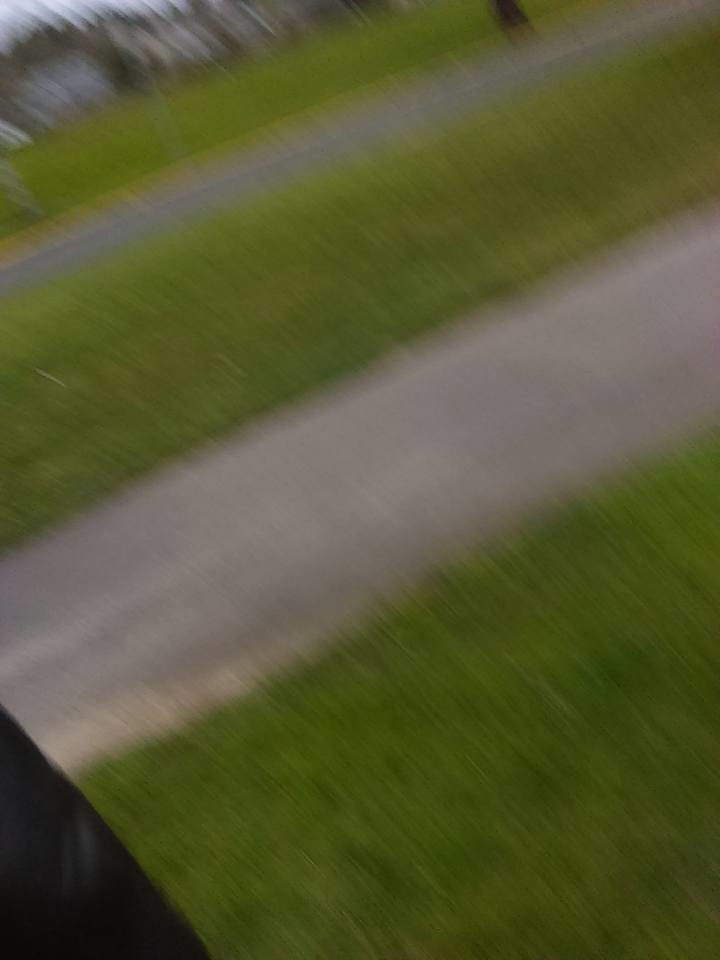The image is a blurry, daytime photograph likely taken while in motion, possibly from a bridge, capturing a scene comprising two asphalt roads with thick green grass strips in between and on either side. The roads appear to be angled, pointing in the same direction which creates a stripy, textured effect. The top left corner of the image reveals blurry houses and potentially some trees or bushes, contributing to the out-of-focus backdrop. A black or dark blue spot, which might be fabric, appears in the lower left corner. Additionally, there is a black mark in the top right corner. The thick grass between the roads suggests a larger distance between the roads compared to their actual width.